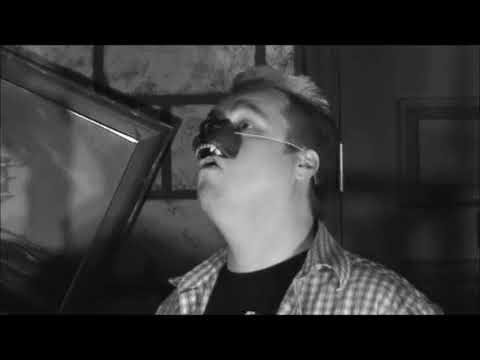The black and white image features a close-up of a man from his shoulders upwards, exuding a playful and goofy demeanor. His amused expression includes wide eyes and a slightly open mouth as he glances towards the upper left. The man sports a rubber werewolf mask, humorously positioned over just his nose with little white teeth visible beneath. The mask's band is noticeable as it wraps around his head. His hair is short, with a mix of dark brown and blonde, some of which sticks up at the top. He wears a black t-shirt beneath a gray and black checkered collared shirt. In the blurred background, there's a tilted picture that resembles a ship, partially obscured, hanging against a brick surface, and a door with silver hinges. The overall scene has a whimsical, almost prank-like atmosphere.